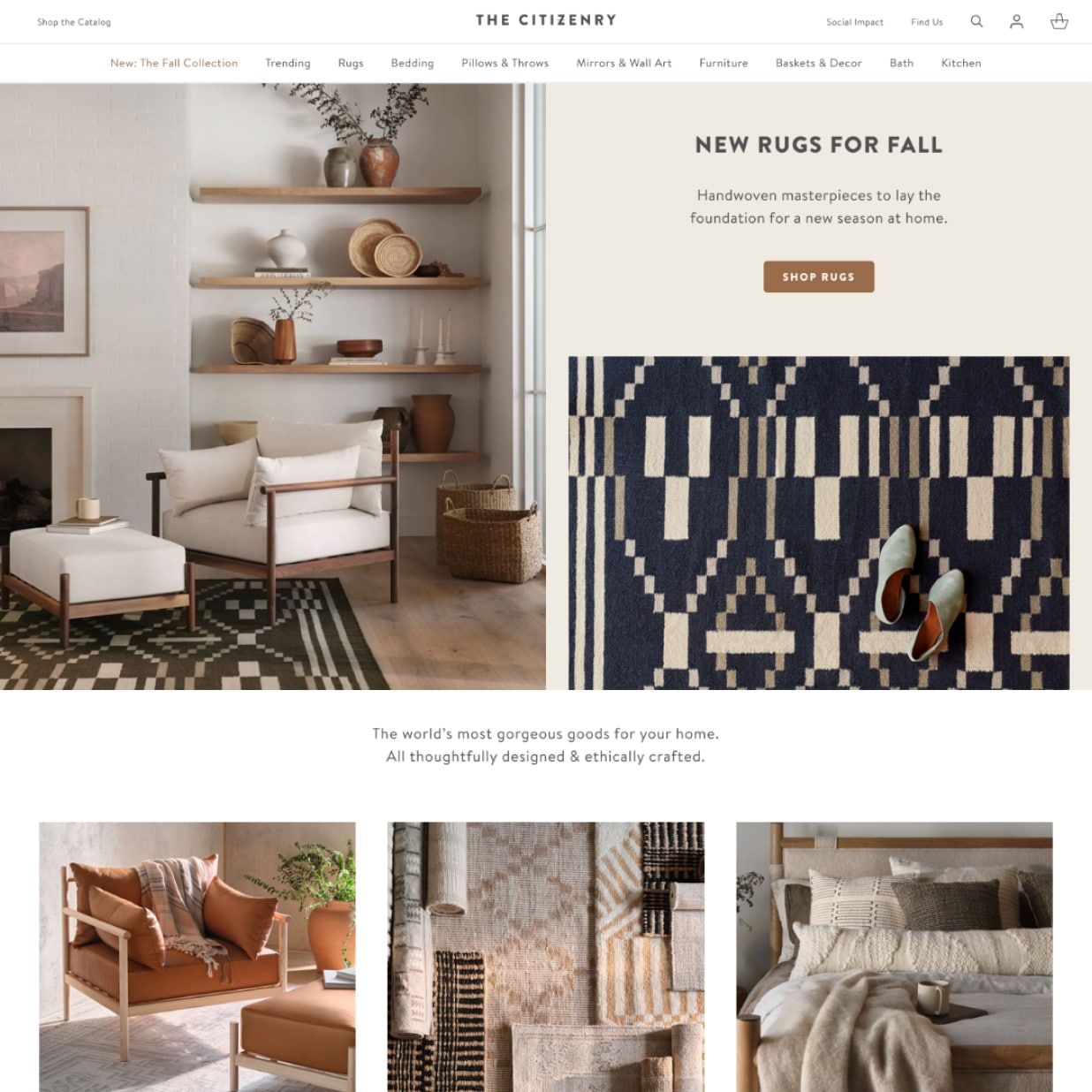At the top of the image, the heading reads "The Citizenry." The top section features a list of categories, though they appear quite blurry. These categories seem to include "Bedding," "Pillows and Throws," "Furniture," "Bath," and "Decor." Further down, the text reads "New Rugs for Fall: Hand-Woven Masterpieces to Lay the Foundation for a New Season at Home." Below this text, a brown button labeled "Shop Rugs" is visible.

The image prominently features a dark blue rug adorned with white square patterns. A pair of shoes is placed on top of the rug. Beneath this, there is a depiction of a bed. To the left of the bed, a close-up of some rugs is shown. Further to the left, another image displays a two-seater chair, which is accessorized with throw pillows and a blanket, enhancing its cozy appearance.